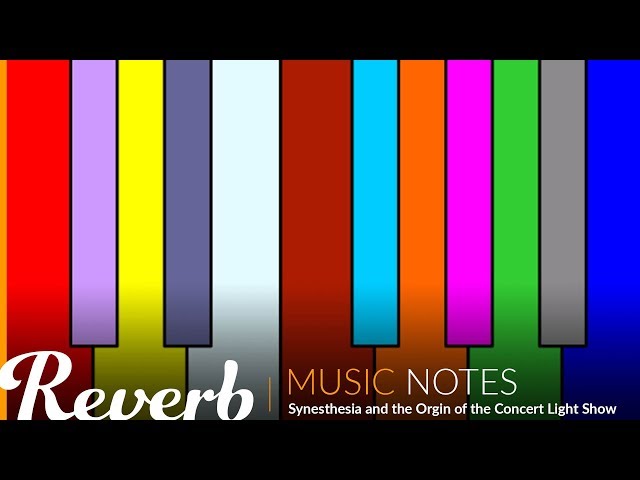This horizontally oriented image features a flat, simplistic, and colorful design of piano keys that appear either hand-drawn or computer-generated. The piano keys are depicted in an array of vibrant colors, including red, lavender, yellow, taupe, white, burgundy, light blue, orange, pink, green, gray, and blue. These colors alternate between larger and smaller keys, representing the familiar layout of a piano but in a visually striking and artful manner.

A black bar frames the top and bottom of the image, giving it a distinct, bordered look. At the bottom of the image, text in various colors and fonts reads: "Reverb" in white on the bottom left, "Music" in orange, and "Notes" in white to the right. Further down, in white font, it reads "Synthesia, and the origin of the concert light show."

This image serves as promotional material, likely a poster or advertisement, with its artistic representation of piano keys and noteworthy typography emphasizing the themes of music and light, suggesting an event or presentation related to the interplay of sound and visual art.